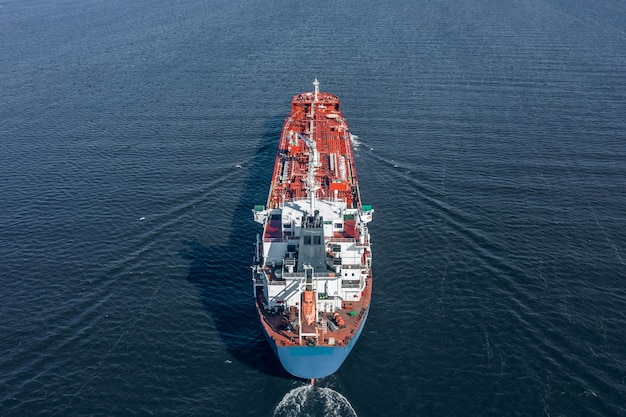This image depicts a large cargo ship navigating a vast, dark blue, possibly greenish body of water, with no land visible on the horizon, suggesting it could be either an expansive lake or the open ocean. The ship, viewed from an aerial perspective, has a reddish-brown deck and a distinct white superstructure, which likely serves as the navigational area and stands several stories high. Towards the stern, the hull transitions to a blue color. The water around the vessel is calm, creating subtle ripples that fan out to the left and right of the ship, indicating its slow movement. Scattered across the deck are various small, indistinct items in colors such as green, red, and white, which might be containers or other cargo. The sun shines brightly, casting a shadow of the ship on the water's left side, enhancing the tranquil yet industrious scene.